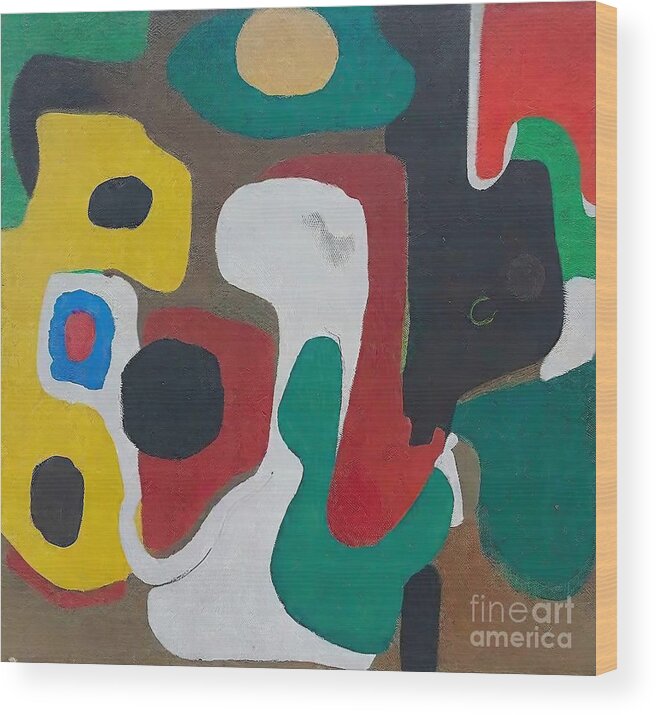This image is a detailed close-up of an unframed abstract painting on a small, square canvas. The painting, which is slightly tilted, features an array of bright colors including teals, tans, yellows, blacks, whites, reds, and blues. The edge of the canvas, which is visible on the right side, is light tan with an orange-brown hue. The artwork consists of various organic splotches and blob-shaped forms that layer and intersect without blending, such as a notable blue area with a red splotch in its center, and a yellow section with solid black circles that resemble the shape of a dog's head pointed downward. The background predominantly appears to be lighter and darker shades of brown. In the bottom right corner of the canvas is the subtle text "Fine Art America."